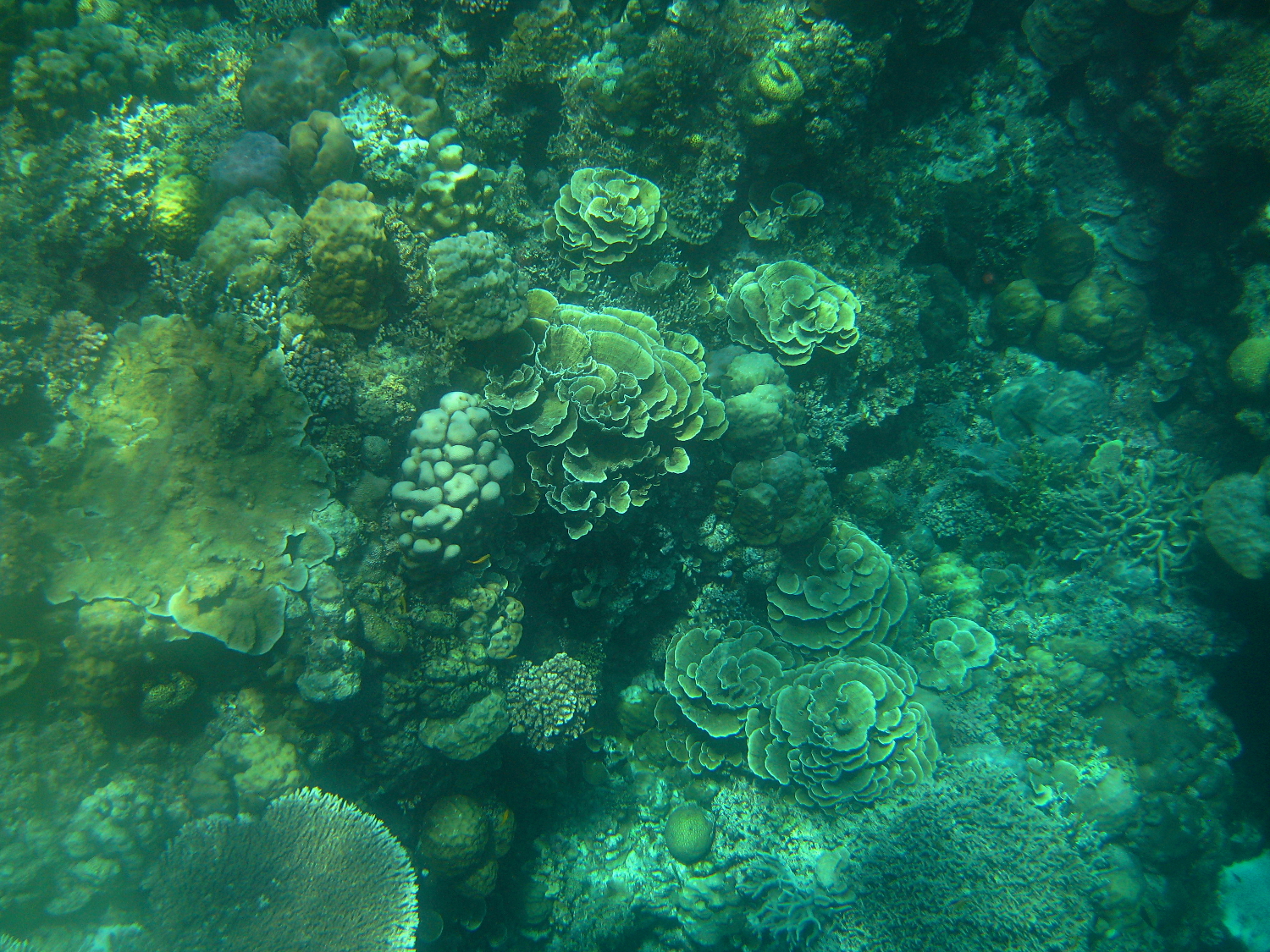The photograph captures a serene underwater scene, dominated by a soothing green hue with hints of teal, yellow, and blue. It depicts a rich marine landscape that could be the floor of a kelp forest or an algae-covered coral reef. Various aquatic plants and corals, some resembling leafy underwater vegetation and round, stacked forms, blanket the environment. There are distinct sections featuring shades of white, yellow, tan, beige, gray, and even black rocks, contributing to the murky greenish-blue water's overall tone. The image evokes a calming underwater ambiance, despite the lack of fish or bubbles, presenting a tranquil snapshot of marine life.